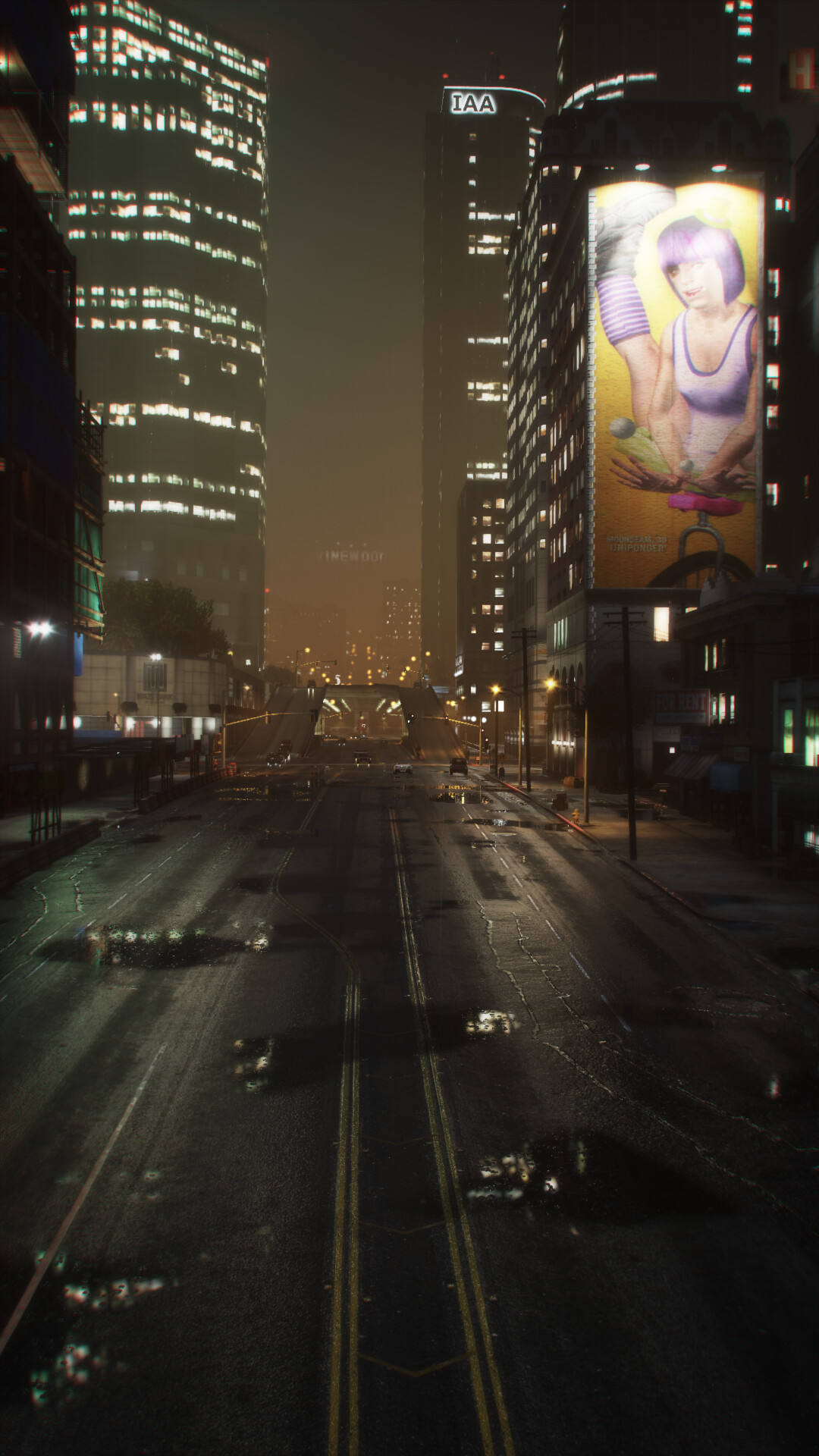This image is an impressive piece of hyper-realistic digital art or a screen capture from a video game, depicting a city street scene at night. The perspective is from a slightly elevated viewpoint, looking down a street that extends from the bottom of the image all the way to the distant background, where the sky appears black with a faint orangish hue along the horizon. Flanking the street are tall skyscrapers, some of which have illuminated windows.

On the left, a large building towers from the ground up. The right side also features a significant structure with a distinct rectangular billboard illuminated by two lights from above. This billboard showcases an Asian woman with purple hair, dressed in a white outfit, seemingly preparing food at a table. Another notable feature on this building is a large advertisement depicting a female in a purple bodysuit and boots, striking a dynamic pose with one leg raised high.

The street itself is a wide six-lane road, marked by two double yellow lines that guide the viewer's eye towards the center of the image and into the depth of the cityscape. Sparse and indistinct vehicles occupy the road, appearing as black blobs without much detail. The scene lacks any visible text or signs, except for the initials "IAA" at the top of the right-center building, adding to the city's mysterious and somewhat futuristic atmosphere.